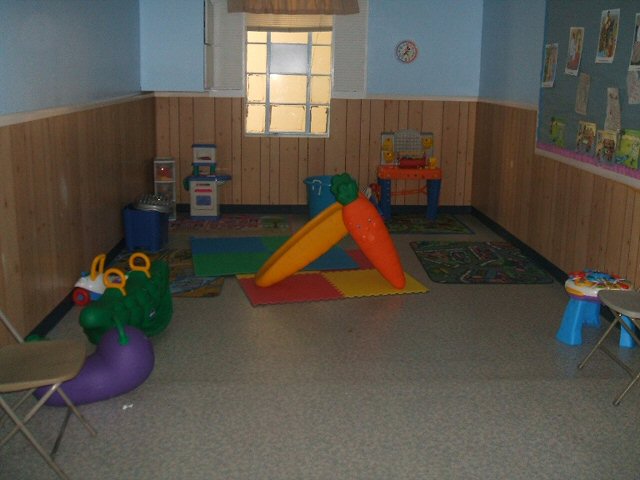The photograph depicts a small children's playroom or classroom, likely designed for kindergartners or preschoolers. The room features a mottled gray concrete floor and light blue walls that transition into light brown wood paneling halfway down. Dominating the central area is a unique small plastic slide with a yellow chute on the left and an orange cartoon carrot base on the right, complete with green leaves where children can step to climb up. Surrounding the slide are colorful padded squares for safety, and a various array of toys are scattered throughout the room. 

To the left, there is a large purple eggplant toy designed for bouncing. Nearby are white and blue ride-on toys, one resembling a car, and several foldable gray seats. The right side of the room features a bulletin board with a dark blue background filled with indiscernible images and clippings, and the back wall hosts a window with white trim and panes partially painted, alongside a clock. Scattered throughout are toys for imaginative play like a pretend kitchen and a tool set, enhancing the room's playful and educational atmosphere.